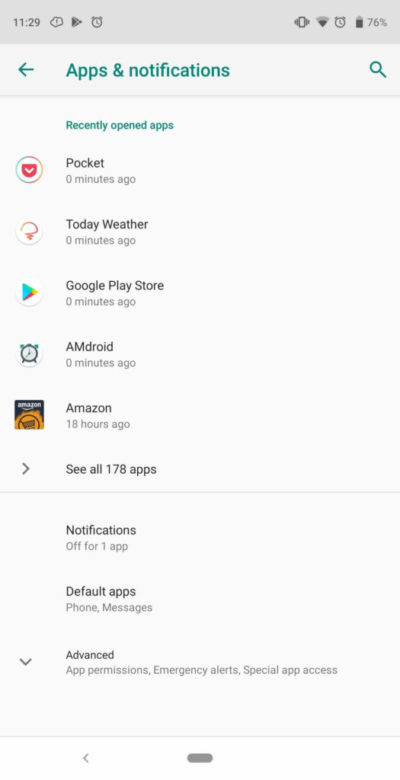The image is a screenshot from a smartphone displaying the "Apps and Notifications" page. The background color is white with a silver-gray border at the top. On the top left corner, the time reads 11:29, while on the top right corner, the battery icon shows a 76% charge. Next to the battery icon, there are symbols indicating an active alarm clock, Wi-Fi connection, and that the phone is on mute. 

Below this, in light green font, is the header "Apps and Notifications," accompanied by a left-pointing arrow on the left side and a search icon (a magnifying glass) on the right. Under the header, the section "Recently Opened Apps" lists the following apps:

- Pocket: 0 minutes ago
- Today Weather: 0 minutes ago
- Google Play Store: 0 minutes ago
- A.M. Droid (alarm clock): 0 minutes ago
- Amazon: 18 hours ago

Following the list, there is an option labeled "See All 178 Apps." Under a thin gray line, additional options are displayed:

- Notifications: off for one app
- Default apps: Phone, Message
- Advanced: App Permissions, Emergency Alerts, Special App Access.